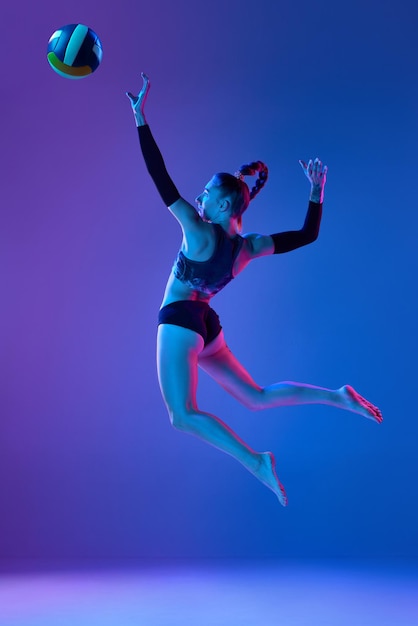The image captures a dynamic moment of a female volleyball player mid-air, about to spike a volleyball. She is airborne with her left hand reaching up towards a blue, white, and yellow volleyball, while her right arm is drawn back. She sports a striking outfit comprising a multicolored sports bra and black bottoms, resembling a two-piece athletic uniform similar to swimwear. Her upper arms are adorned with black arm sleeves or bands. Her hair, braided atop her head and swinging out in a ponytail, adds to the sense of movement. The background features a vivid blend of purplish-blue hues, blurred to enhance the focus on her action, with lighting effects casting subtle blue and pink tones across the scene. Her posture is energetic, with legs bent and extended behind her, encapsulating the intensity and grace of the sport.